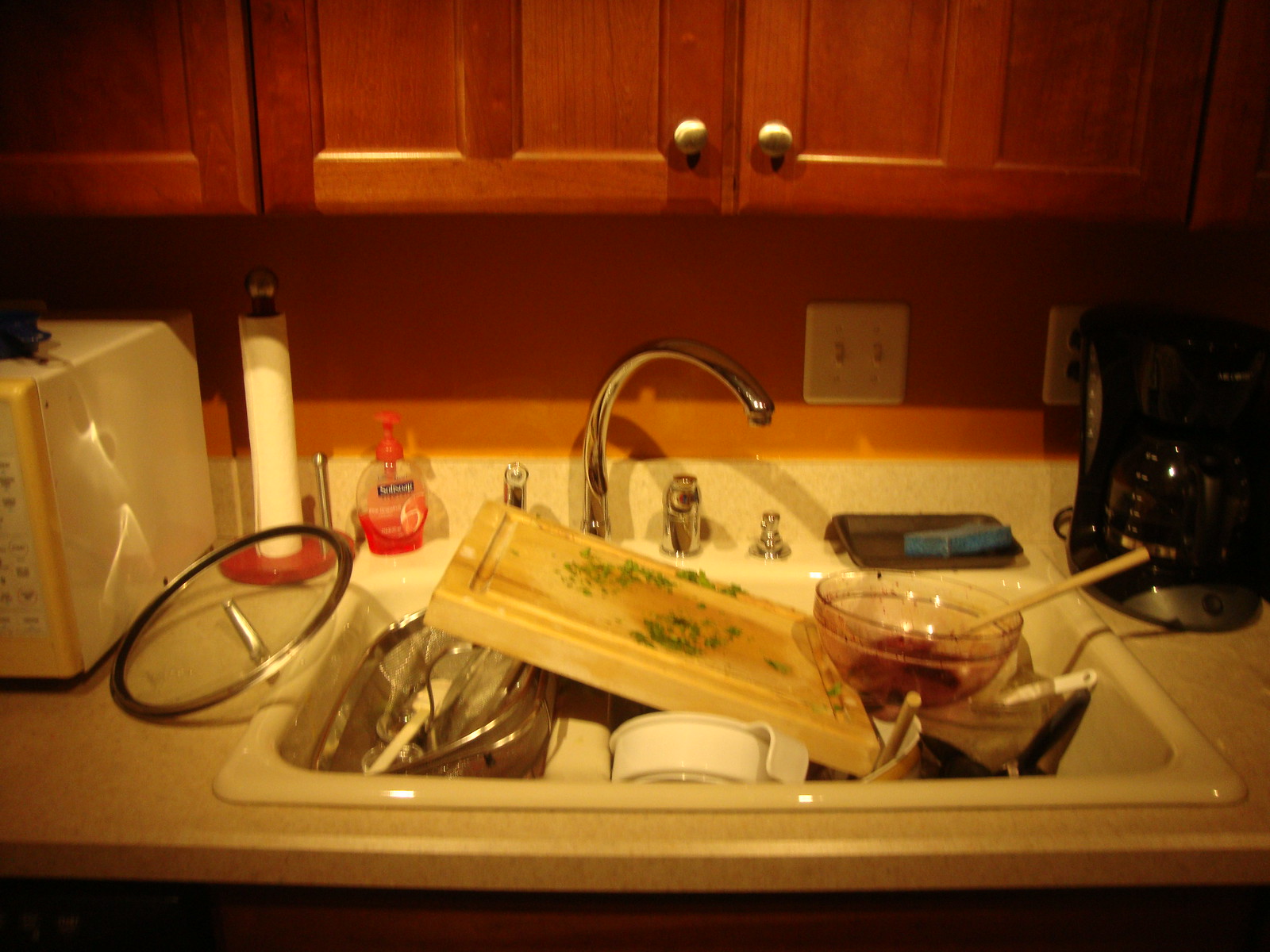A cluttered kitchen scene captures a sink filled to the brim with dirty dishes, suggesting a recent bout of extensive cooking. Atop the precarious pile sits a cutting board, which holds a glass bowl at its base with a wooden spoon jutting out, hinting at unfinished culinary tasks. Concealed beneath the cutting board are larger, indistinct metal items, the remnants of a busy kitchen session. The sink is set into an off-white countertop and features sleek chrome fixtures. Adding warmth to the setting, the wall behind the sink is painted a burnt orange, harmonizing with the wood-toned cabinets above, each equipped with nickel-colored knobs. Flanking the sink are practical kitchen accessories: a coffee maker to the right and, on the left, a paper towel holder beside the edge of a microwave that just enters the frame. The scene illustrates the aftermath of an industrious cook at work, set against a backdrop of functional yet stylish kitchen decor.